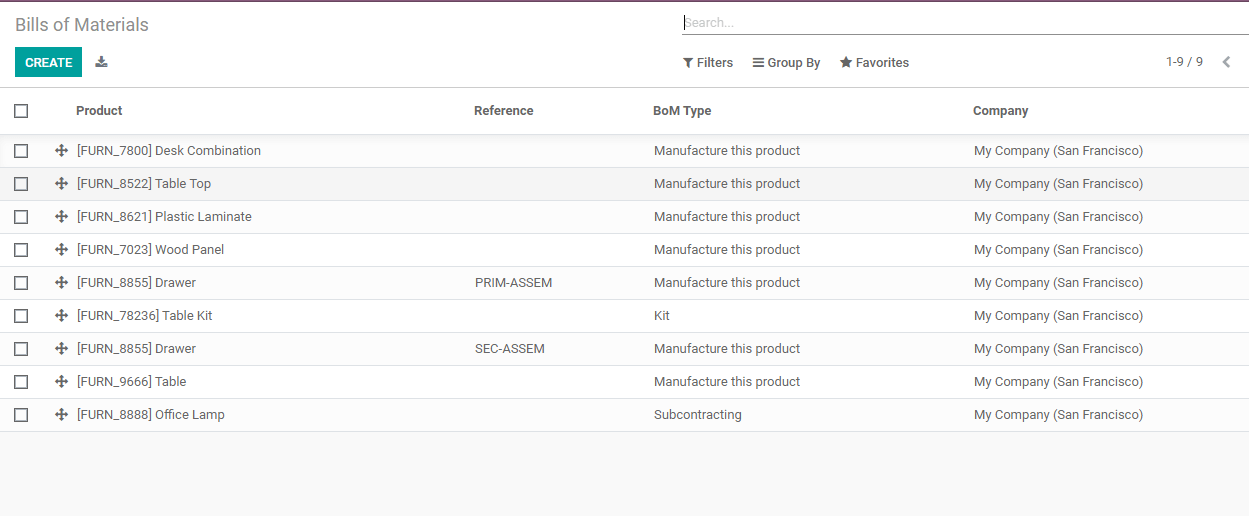The image depicts a formal Bill of Materials (BOM) list located in the top left corner. The BOM is presented as a structured table with a minimum of four columns. Each entry in the list is categorized under the header "FURN" (in all caps), followed by the specific item type, such as desk combination, tabletop, plastic laminate, wood panel, drawer, cable kit, table, and office lamp. 

Notably, the table does not include any pricing information, suggesting that the document is intended for business-to-business transactions, possibly detailing office furniture specifications. The columns in the table are labeled as "Reference," "BOM Type," and "Company." The "BOM Type" column predominantly contains the term "manufacture this product," while the "Company" column simply states "My Company, San Francisco." The "Reference" column is mostly empty, except for a few cryptic entries like "SEC-ASSEN."

Additionally, there is a search bar positioned at the top of the image, potentially indicating that this BOM is part of a digital interface or software designed for inventory management or procurement.